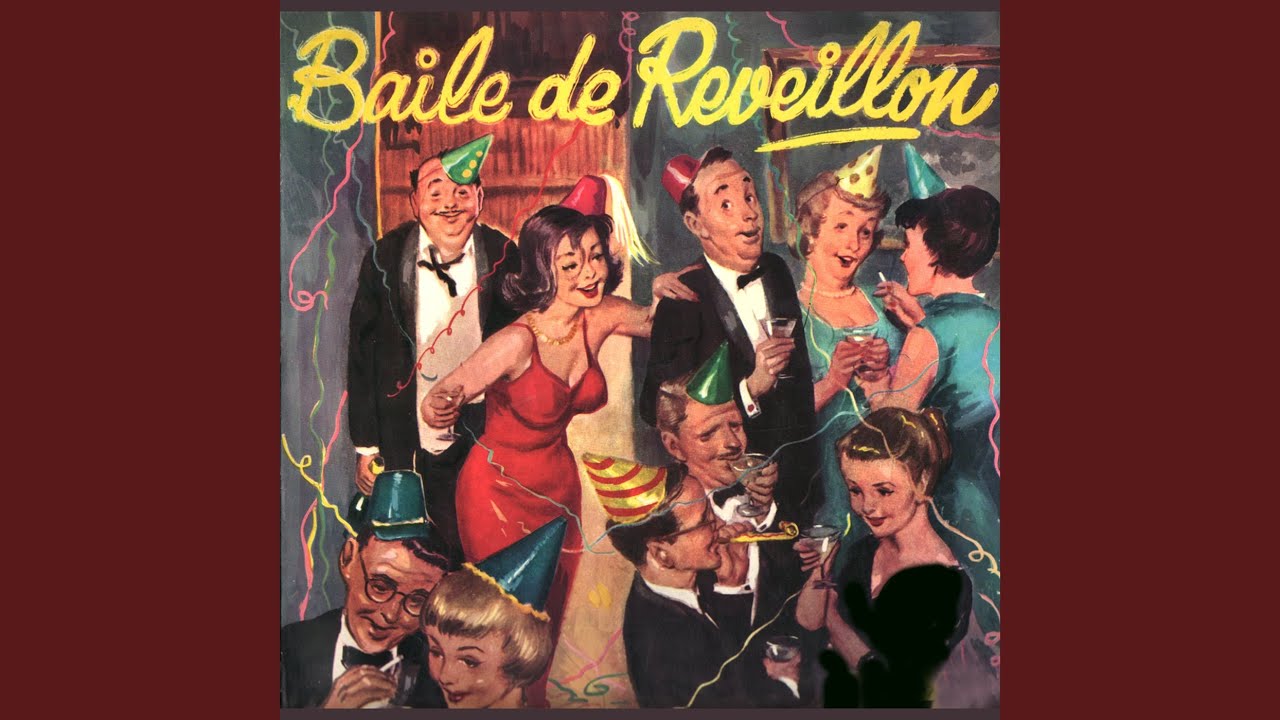This image, titled "Ballet de Reveillon" in bright yellow cursive at the top, seems to be an advertisement or possibly an album cover from the late 1960s. It features a lively party scene with a mix of men and women, all dressed in formal attire—men in black and white tuxedos and women in colorful dresses, including red, blue-green, and black. Party hats are a common accessory, ranging from pointy cone hats to colorful fezes, adorned with tassels and other festive details.

At the heart of the image is a prominent woman in a strapless red dress. She stands slightly left of center, holding a glass of champagne in her right hand, her left hand resting on the shoulder of a man beside her who is also in a suit and holding a drink. The party atmosphere is vibrant, with streamers and confetti airborne, suggesting an ongoing celebration akin to New Year's Eve.

The setting appears to be indoors, possibly a living room or a library, indicated by the presence of bookshelves in the background. Among the other festive details, some guests are seen smoking or sipping on martinis while others engage in conversation or blowing on party favors. The overall mood is captured by the cheerful expressions and dynamic interactions among the party-goers, capturing a sense of relaxed yet spirited enjoyment.